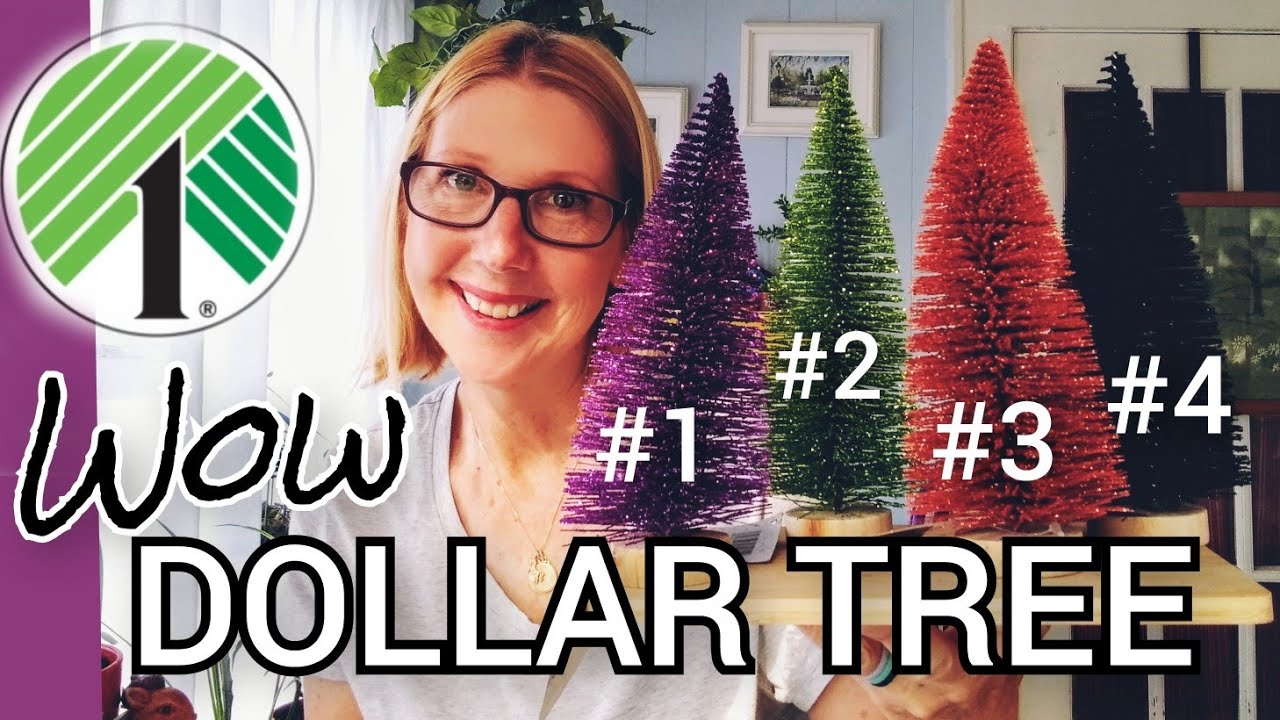This vibrant and festive social media graphic features a cheerful woman standing in her cozy living room, where the blue walls add to the inviting atmosphere. She is holding a wooden tray with four small, decorative tinsel Christmas trees in different colors: a purple tree labeled "1," a green tree labeled "2," a red tree labeled "3," and a black tree labeled "4." Her long blonde hair frames her face, and she peers through black-framed glasses with a delighted smile directed at the camera.

In the top left corner, the Dollar Tree logo is prominently displayed, accompanied by a black number "1" inside a circle. Below the logo, the word "WOW" stands out in large black letters, followed by "Dollar Tree" in bold, white letters with black outlines across the bottom of the graphic. This eye-catching caption emphasizes the affordability and variety of festive decor available at Dollar Tree, as showcased by the influencer.